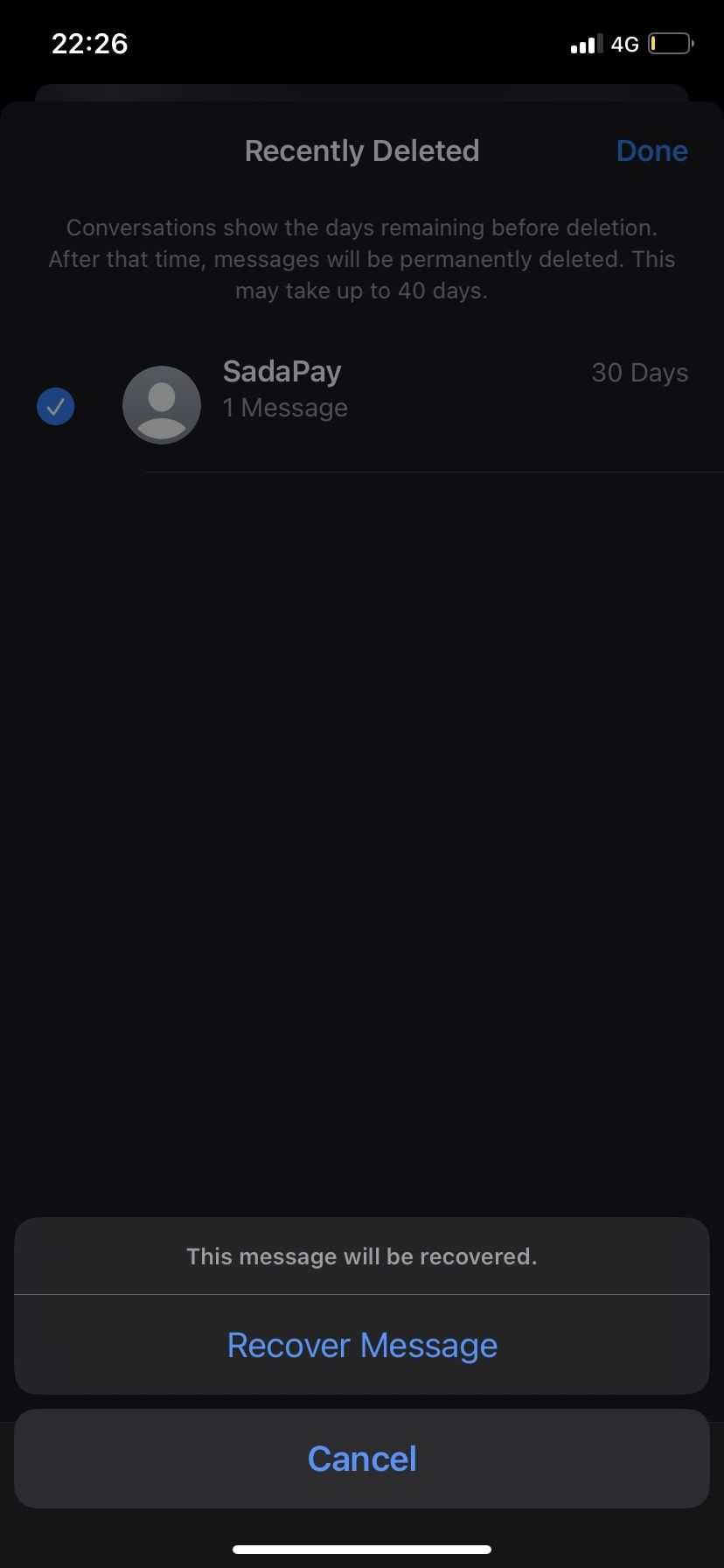The image depicts a cell phone screen captured at the time 22:26, as indicated in the upper left-hand corner. The device boasts a strong signal connection and is operating on a 4G network. However, the battery life is critically low, with the battery icon nearly depleted.

The screen shows a section labeled "Recently Deleted" in light gray text against a black background. Beneath this header, there is a notice explaining that conversations displayed here will be permanently deleted after a certain period. The text, which is faint and challenging to read, states: "Conversations show the days remaining before deletion. After that time, messages will be permanently deleted. This may take up to 40 days."

Immediately below the notice, there is a specific deleted conversation from a contact named "SATA pay," which is represented by a generic gray avatar icon. This contact has one message associated with it. To the right of the contact's name and message count, there is a round blue circle with a check mark, labeled "30 days," indicating the time remaining before the message is permanently erased.

Further down, there is an option to recover the message, highlighted in blue text that says, "Recover message." Directly underneath this, another blue button offers the option to "Cancel," allowing the user to choose whether or not to save the conversation before it is deleted permanently.